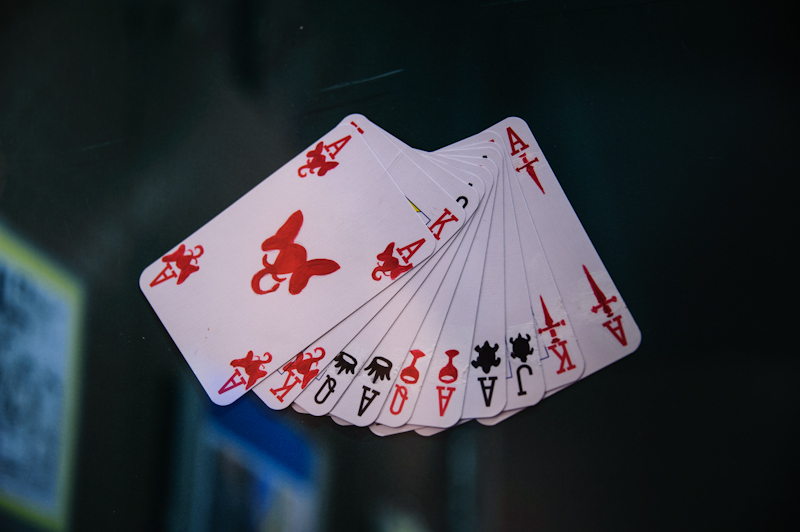The image showcases an assortment of what appear to be handmade playing cards, each featuring unique and imaginative designs rather than the traditional suits. The cards are either suspended or taped, creating a dangling effect against a backdrop that looks like an outdoor scene viewed through a window.

At the forefront is an intricately designed Ace of Elephants card. The card, placed diagonally in the photo, features a prominent red elephant head in the center. The corners of the card display two A's accompanied by smaller elephant heads at the top, and two upside-down A's with elephant heads at the bottom.

Fan-like behind it is a King of Elephants card. Only an upside-down K with an elephant is visible, with the right-side-up K peeking from behind. The next visible card is a Queen, depicted in black with a crown, also seen upside down. This is followed by a black Ace adorned with a crown.

Continuing along, the sequence reveals a red Queen holding a wine glass, a red Ace with a wine glass, a black Ace featuring a turtle, and a black Jack with a turtle motif. The penultimate card is a red King brandishing a sword or dagger, and the assortment concludes with an Ace displaying a downward-pointing dagger, mirrored at both the bottom and top corners of the card.